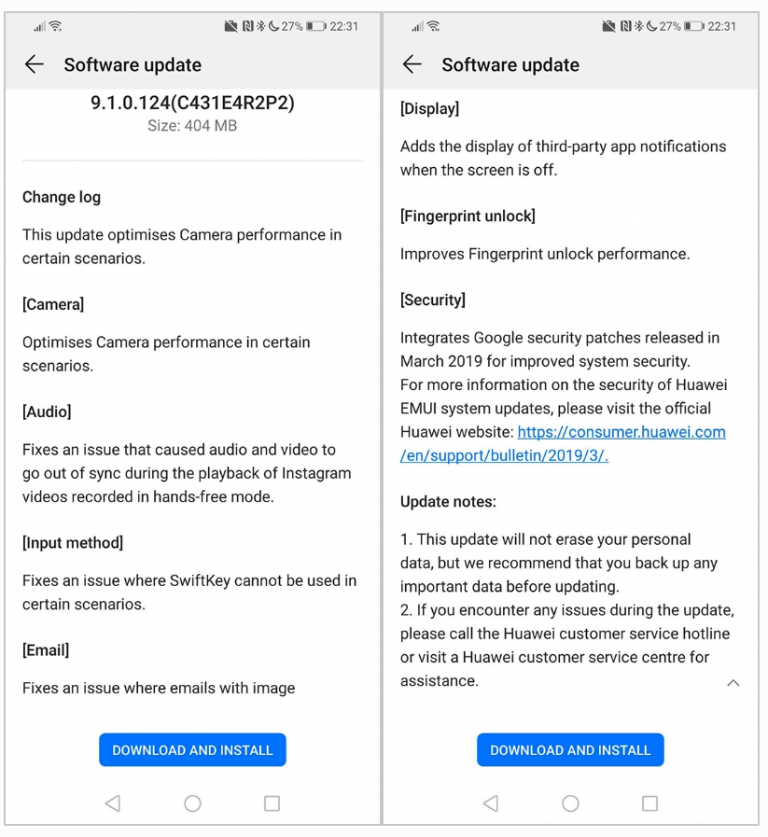In this image, there are two screenshots displaying the software update settings page on a mobile device.

**Screenshot on the Left:**
- The top of the screen features a typical mobile gray border, showing the Wi-Fi signal and battery icon.
- Below this border, the header "Software Update" appears in black, with a left-facing arrow for navigation.
- The main content area has a white background.
  - At the top, it displays the update version "9.1.0.124" with the identifier "(C431E4R2P2)" beneath it in black text.
  - The update's size, "404MB," is mentioned in gray font.
  - Below, a faint gray separator line divides the content.
  - Several update items are listed:
    - **Change Log:** Indicates improvements and fixes:
      - **Camera:** "Optimizes camera performance in certain scenarios."
      - **Audio:** "Fixes an issue that caused audio and video to go out of sync during the playback of Instagram videos recorded in hands-free mode."
      - **Input Method:** "Fixes an issue where switch key cannot be used in certain scenarios."
      - **Email:** "Fixes an issue where emails with image..."
  - At the bottom, a blue rectangular button labeled "Download and Install" in white text is present.
  - The navigation menu at the bottom has three icons: a left-facing play button, a circle, and a square.

**Screenshot on the Right:**
- It has a similar layout with the gray border at the top, Wi-Fi, and battery indicators.
- The header "Software Update" and the back arrow are consistent with the first screenshot.
- The update details continue on a white background:
  - **Display:** "Allows display of third-party app notifications when the screen is off."
  - **Fingerprint Unlock:** "Improves fingerprint unlock performance."
  - **Security:** "Integrates Google security patches released in March 2019 for improved security. For more information on the security of Huawei EMUI system updates, please visit the official Huawei website (https://consumer.huawei.com)."
  - **Update Notes:**
    - "This update will not erase your personal data, but we recommend that you back up any important data before updating."
    - "If you encounter any issues during the update, please call the Huawei customer service hotline or visit a Huawei customer service center for assistance."
  - Like the left screenshot, a blue button labeled "Download and Install" is at the bottom.
  - The bottom navigation replicates the icons seen in the first screenshot: left-facing play button, circle, and square.

These screenshots comprehensively show the software update details, new features, issues fixed, and instructions for installation on the mobile device.